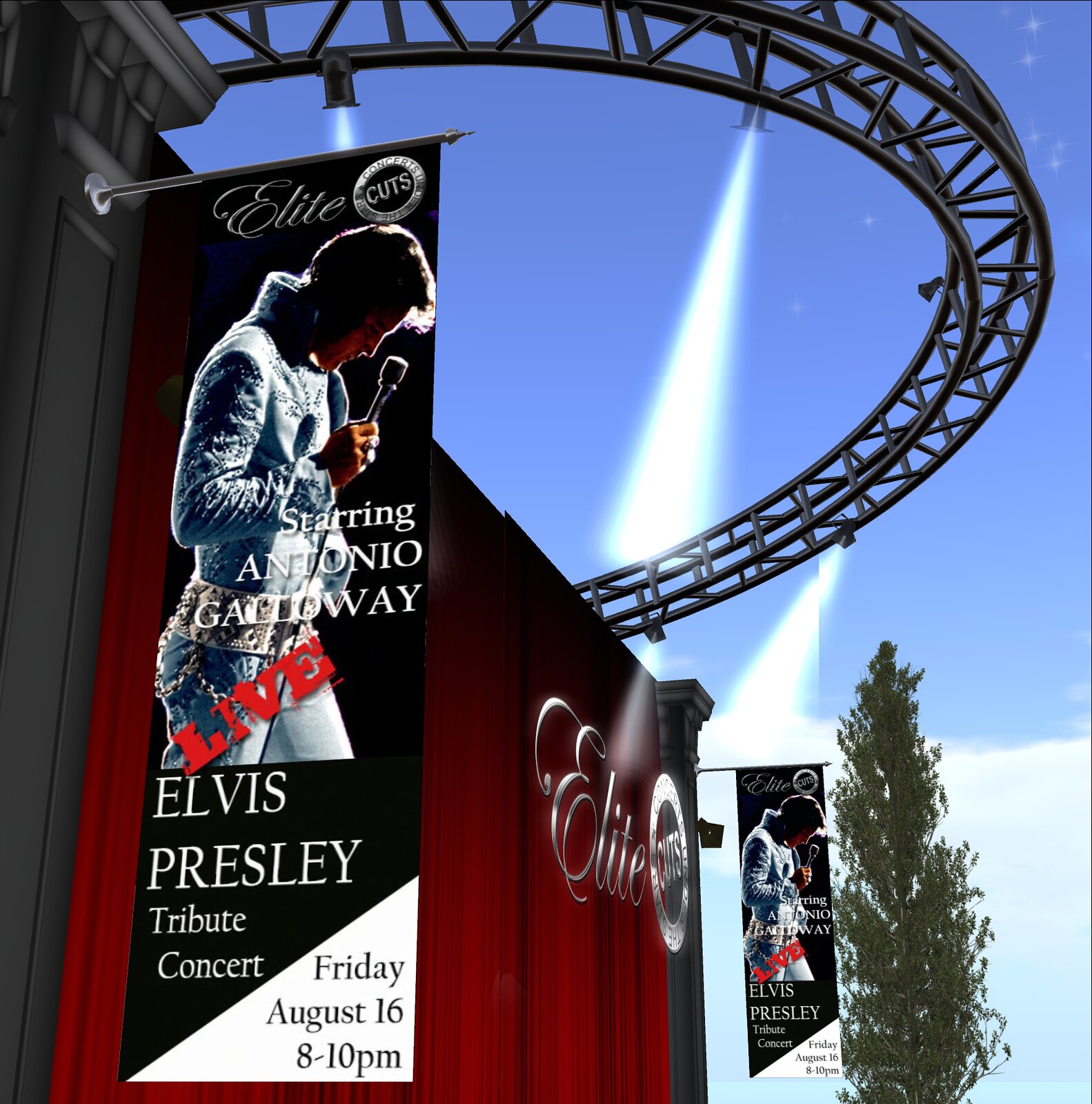The image depicts a 3D rendering of a concert hall, designed to visualize the setup before its real-life construction. Situated on the left-hand side of the image is a stage adorned with long red curtains and supported by gray pillars. A notable architectural feature is the metal semicircular element that spans across both sides of the building. Above, the sky and trees add to the background ambiance of the scene.

Prominently displayed are two identical signs, each featuring a prominent picture of Elvis Presley holding a microphone and gazing downwards. Elvis is dressed in a very silvery, shiny outfit complete with a matching belt. The sign reads "Elite" at the top, accompanied by the headline, "Starring Antonio Galloway." It also announces in bold red letters "Live" and includes the details "Elvis Presley Tribute Concert" in white letters. The event is scheduled for "Friday, August 16th, 8 to 10 p.m.," written in black letters. The meticulous detail of the signs contrasts with the overall rendering's video game-like feel, emphasizing their official design despite the pre-construction visualization setting.